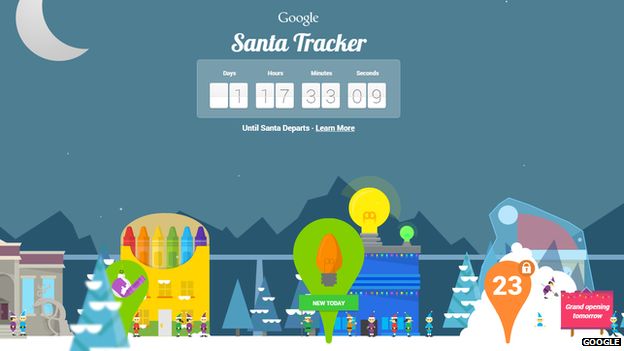In this image, a festive Christmas-themed screenshot from Google's Santa Tracker page is prominently displayed. At the very top, the familiar Google logo confirms its origin. The main focus is the countdown timer for Santa's departure, presented in white text against a vividly designed backdrop, emphasizing the holiday spirit.

The title "Santa Tracker" is clearly visible, although the image is slightly blurry. The countdown is broken down into days, hours, minutes, and seconds, currently showing 1 day, 17 hours, 33 minutes, and 9 seconds remaining until Santa departs—indicating the current date is likely December 23rd. Below the countdown, the phrase "until Santa departs" further clarifies the timer's purpose, inciting excitement for the upcoming Christmas Eve.

A "Learn More" link is also present, inviting users to explore further details about the Santa Tracker event. The overall design of the page is cheerful and child-friendly, featuring various Christmas-themed elements that enhance its festive appeal. The top section of the page is relatively small, highlighting the tracker. The bottom section, however, boasts a rich array of holiday graphics: a pack of crayons, colorful light bulbs, a glacier, snow-covered trees, and buildings in the foreground. The background showcases an outline of majestic mountains, completing the charming winter scene.